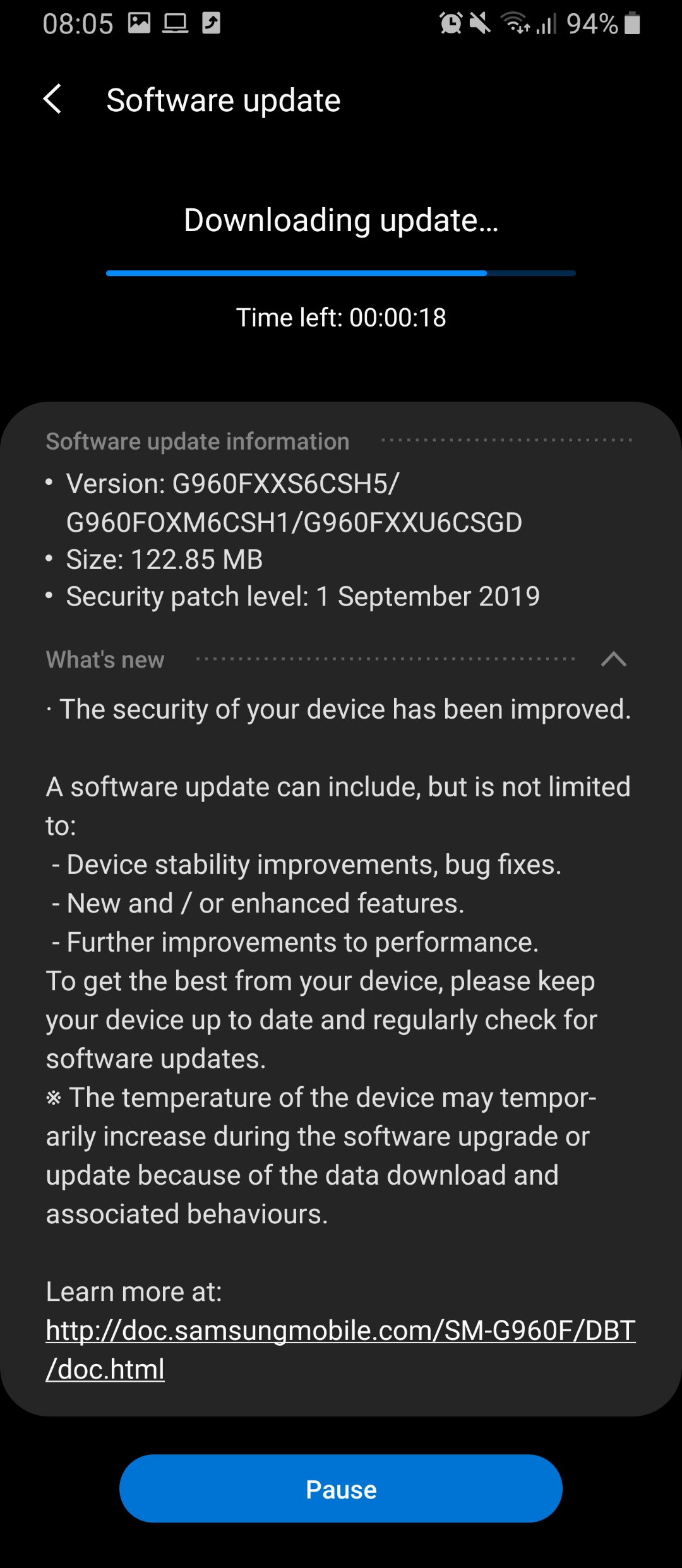Screenshot of a software update page, featuring the following details: At the top left, the header reads "Software Update." Below this, there is a progress indicator that states "Downloading update," with 18 seconds remaining. The section titled "Software Update Information" lists the version number as a lengthy string, followed by the file size of 122.85 MB. Additionally, the security patch level is dated 1 September 2019. The "What's New" section notes that "The security of your device has been improved." The image also includes supplementary information such as the current temperature of the device and a tip advising users how to maintain their device's updates.